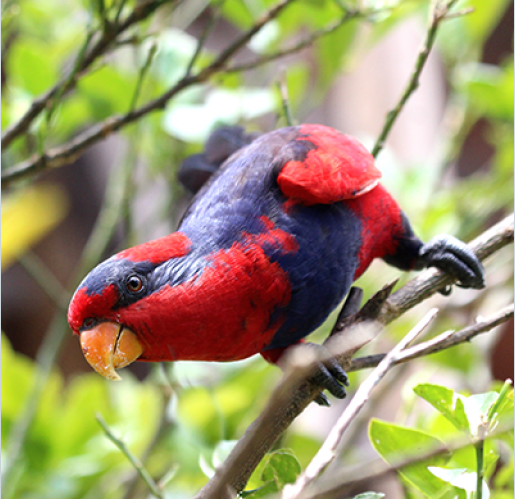This vibrant photograph captures the striking detail of a small tropical parrot, specifically a red and blue lorry, perched on a thin, brown tree branch. The bird's colorful plumage is distinctly divided: its head is predominantly red, with the vibrant hue extending under its beak, along its chest, and on the back portion of its head. The rest of its body, including its belly and back, has a rich, dark blue color that contrasts beautifully. Its yellow-orange beak and dark brown eye add to this intricate color palette. The bird's talons, which are black, grip the branch firmly, showcasing its elegant, yet composed stance. The parrot's orientation is unique, as it leans forward at a 45-degree angle, with its head pointed downward to the left corner of the image, giving an impression of it almost being upside down. Surrounding the bird is a lush environment with green leaves and out-of-focus branches, highlighting the bird as the photo's primary subject. The background, slightly blurred, emphasizes the parrot's vibrant colors and textures, making this photograph a mesmerizing display of tropical wildlife.